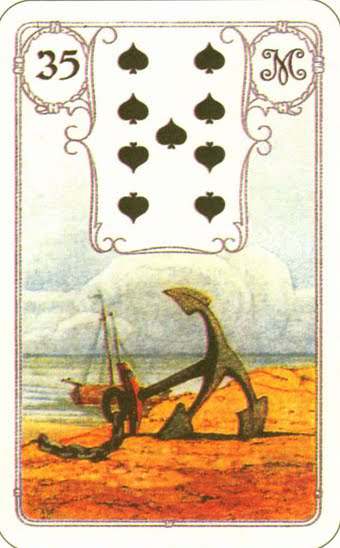The image is an intricate drawing of a decorative card. In the top left corner, there is a circular emblem outlined with a rope-like ring, and inside the circle, it is filled with black, prominently displaying the number "35." To the right of this emblem, there's a depiction of a person encircled by a ring.

At the center of the card, there is a smaller card-like shape, bordered intricately at each corner—top left, top right, bottom left, and bottom right. Flanking this central card are four spades on each side. In the very center of this setup, there is also a single spade.

Below this central arrangement, the illustration transitions into a serene beach scene. The background showcases a blue sky dotted with mostly white clouds. Stretching across the horizon is a calm expanse of water. A large ship with a brown hull and a prominent mast with strings extends upwards, adding a touch of maritime adventure to the scene.

The foreground features sand dominating the landscape, with some patches of brown dirt. At the very bottom, there's a depiction of chains connecting to an anchor. The anchor has a round hole in the middle, with its design extending laterally and vertically. It comprises hooks: one extending up, another long hook extending to the left, and the third hook pointing down to the right, with two of these hooks embedded in the ground and one pointing upwards into the air.